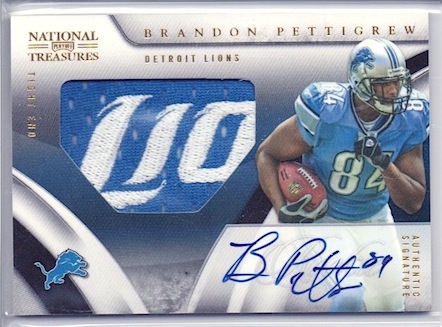The image depicts a detailed sports trading card from the National Treasures series by Panini, featuring Brandon Pettigrew of the Detroit Lions. The upper left corner showcases the National Treasures logo, while above the player’s image, Brandon Pettigrew's name is printed in gold. The player, a muscular black man, is captured in action, wearing a teal Detroit Lions jersey with the number 84 on his chest, and holding a football under his right arm as he runs. His left arm is bent at the elbow, and he is helmeted. The bottom of the card features an on-card authentic signature signed in blue ink by Pettigrew, including his jersey number 84. There is also a visible patch of his jersey on the card, displaying the letters "LIO" from the word "Lions." The distinctive Detroit Lions logo in bright turquoise blue is present in the lower left corner. The card is predominantly silver and gray in color with a colorful and visually appealing design.